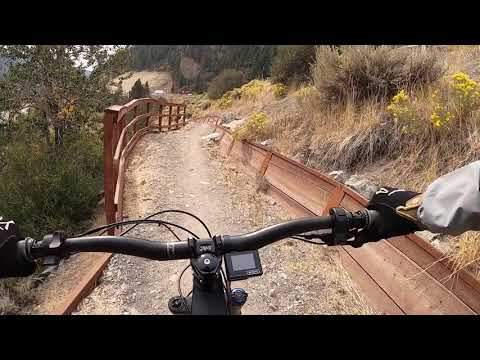The image captures a dynamic view from a mountain biker's helmet-mounted GoPro, as they navigate a narrow dirt trail etched into the side of a hill. The trail is flanked by protective wooden fences on both sides. On the left side, which descends sharply, there is a taller red fence intertwined with bushes and brush, safeguarding the rider from the steep drop. On the right side, the uphill section, there is a shorter, solid brown wooden fence holding back dirt, weeds, and scattered yellow foliage. The biker's black bicycle, equipped with a straight handlebar with a digital display and hand brakes, is clearly visible, showcasing the gripping experience of trail riding. As the path stretches out ahead, patches of pine and deciduous trees can be seen further along, contrasting with the surrounding brown terrain. A camera mounted on the bike's transverse bar points forward, capturing the thrilling descent along the scenic mountain trail.